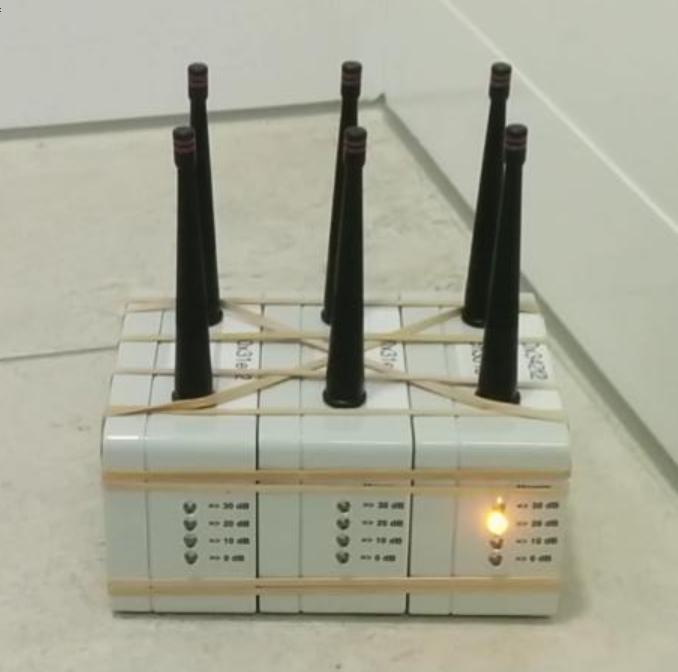The image displays a neatly arranged formation of six white cubes, each equipped with a tall, black, three-inch antenna protruding from the top. Each cube features a vertical row of four LEDs along one side, with one of the cubes showing at least one illuminated LED. The cubes are intricately bound together using several rubber bands wrapped horizontally and diagonally around the group, creating a compact cluster. Although there is some writing on the cubes, its details are obscured due to the picture's angle. The entire assembly rests on a tiled floor, making the sleek, white cubes and their black antennas stand out clearly against the background.